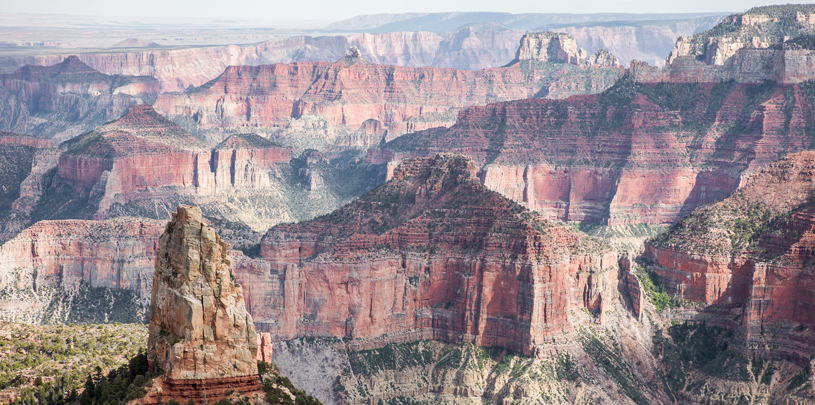This breathtaking aerial view showcases the vast expanse of the Grand Canyon, captured from a lofty vantage point that reveals both its majestic depth and intricate landscape. At the forefront, a prominent rocky outcliff juts upward from the bottom left, standing prominently against the hazy blue sky that stretches across the horizon. The heart of the image is dominated by the multi-layered canyon terrain, characterized by its striking red and rust-colored stone formations, which cascade across the scene from left to right. Sparse vegetation, consisting of hardy flowers, small trees, and greenery, clings to these imposing cliffs, adding bursts of life to the arid landscape. In the bottom left section, a notable structure or monument appears, suggesting a potential gathering spot or overlook designed for visitors to marvel at the natural wonder. The image was taken in daylight, illuminating the subtle textures and vast layers of the canyon, making it a vivid representation of the iconic Grand Canyon.